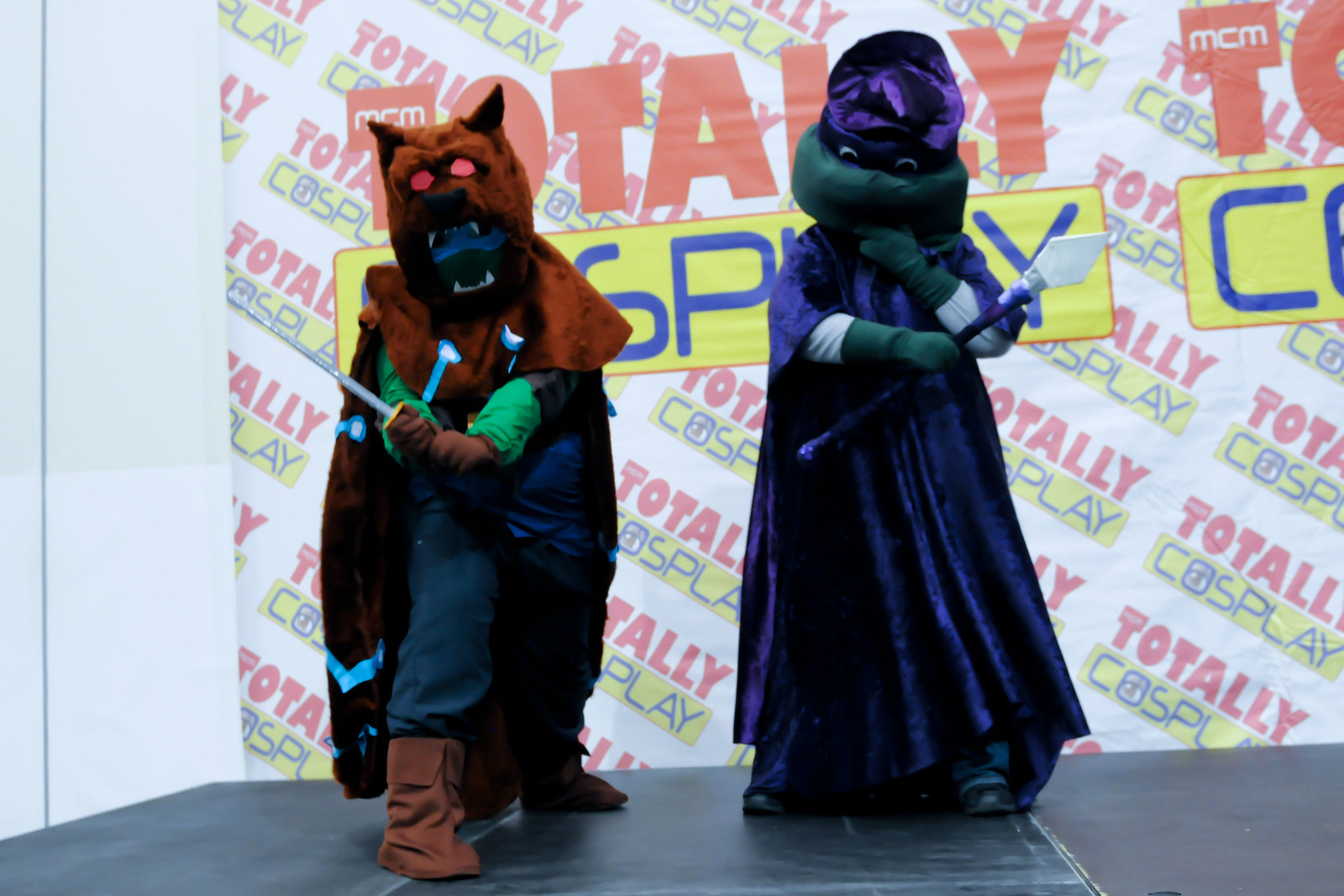In the photo, two individuals are dressed in elaborate costumes, presenting a compelling scene that appears to be from a convention or cosplay event. Both of their faces are obscured by intricately designed masks. The first individual is adorned in a costume that resembles a ferocious creature, possibly a wolf. The mask is brown with intimidating sharp teeth and red eyes, and this person wields a large sword. The second individual is clad in a costume that hints at a fantastical reptilian creature, with a green face evocative of a Teenage Mutant Ninja Turtle. They wear deep purple wizard robes and a matching cap, and they are holding a spear in one hand. The backdrop of the image features a repetitive "Totally Cosplay" display in bold red and blue fonts, accented by a yellow band with an anime eye in the 'O,' solidifying the cosplay event atmosphere.